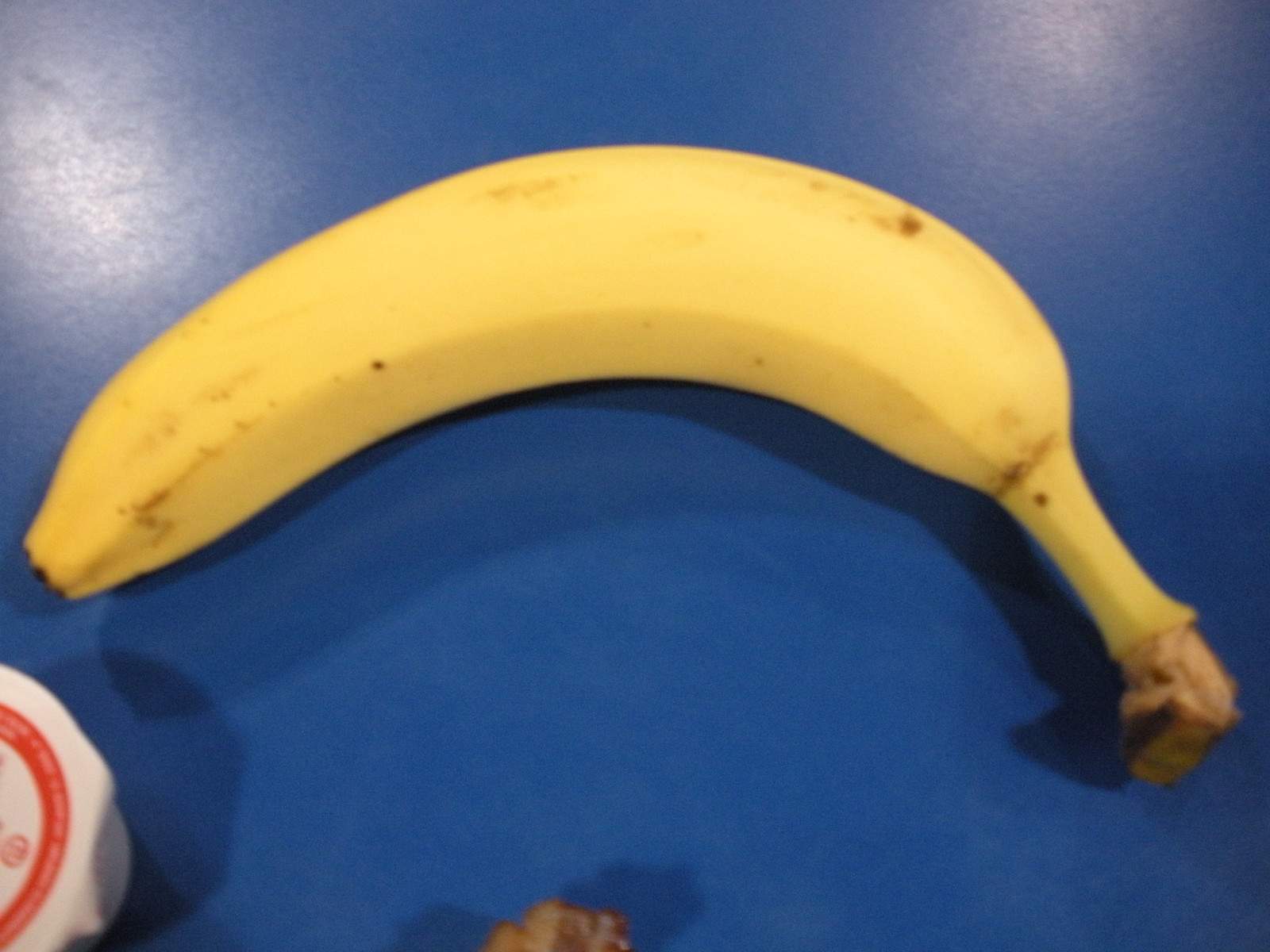This photograph showcases a ripe banana placed on a blue tabletop. The banana is centrally positioned in the image, curving downward in a distinct U-shape. Its tip points to the left mid-center of the frame, while the stem, which would typically be attached to the vine, is located on the right side. The banana has several brown spots, particularly concentrated at the tip, the top quarter, and along the edge of the stem.

In the background, the reflection of two overhead lights is visible. The brighter overhead light is situated in the top left corner, while a dimmer light occupies the top right corner. Additionally, there is a circular object in the bottom left corner; it is white with a red rim and features white lettering. Another unrelated brown object is positioned towards the bottom center of the image.